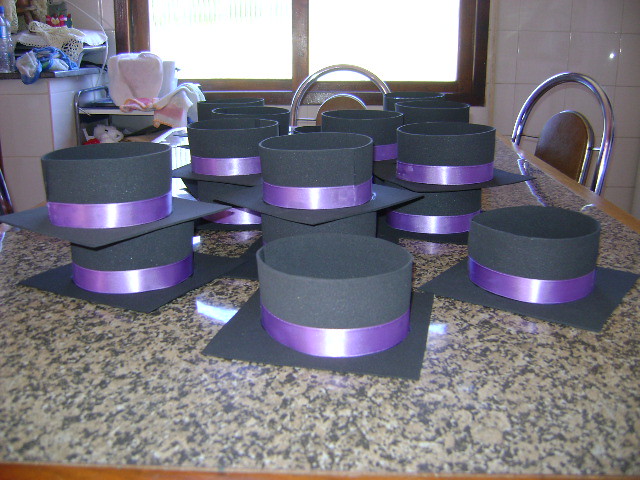In this image, we see what appears to be a collection of handmade, costume-style hats, evoking the design of graduation caps, arranged on a marble-like countertop with black speckles and wood trim. The hats are characterized by their distinctive square base and rounded, raised tops, each adorned with a vibrant purple ribbon encircling the base of the rounded part. The hats are crafted from materials resembling foam, construction paper, or felt, suggesting they are intended for decorative or craft purposes rather than actual wear. The setting appears to be a personal space, likely a home, as evidenced by the background details: shelves with various items, a cabinet displaying lace doilies, blankets, and a teddy bear, and a double window against white-tiled walls. The table, which is possibly being used as a crafting station, has several hats stacked either singly or in pairs, totaling between 20 to 25 hats. Additionally, there are hints of chairs around the table, further indicating it could be a communal or dining area within a home.